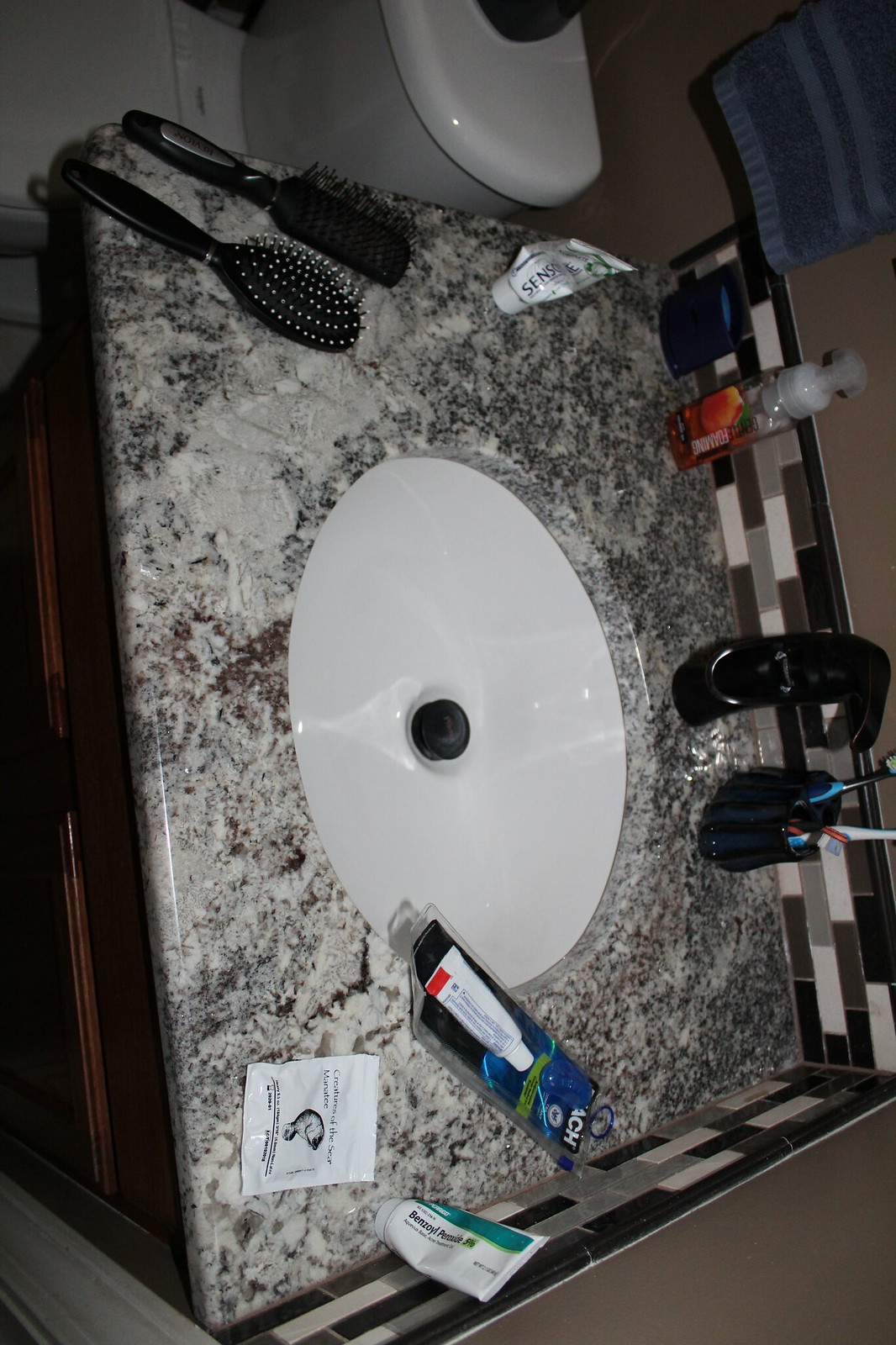The image, a color photograph, is currently rotated 90 degrees to the right and needs to be adjusted 90 degrees to the left for the correct orientation. The poorly lit bathroom scene features a tank and part of the lid of the toilet on the left side, which appears at the top left corner of the sideways image. In the top right corner, part of a blue hand towel with decorative bands hangs visibly. 

The bathroom setup includes a freestanding wooden vanity cabinet with two doors, although the doors are partially cropped out of the image. The vanity top is adorned with a faux granite finish and hosts a seamlessly integrated white sink. A conspicuously busy tile backsplash and side splash feature 1 by 3-inch tiles in a mix of white, black, brown, and tan, extending approximately four rows high, wrapping around the corner of the sink area.

On the countertop, various items are scattered. On the left side, which appears at the top in the current orientation, a foaming pump soap dispenser, potentially from Bath and Body Works, sits next to a toothbrush and toothpaste caddy. A squeezed, nearly empty tube of medicine lies on the right side of the sink, with a small travel-sized toothpaste tube positioned nearby. Adjacent to an arc-shaped faucet, which likely integrates its handle, are two black hairbrushes—one with traditional bristles and another with pin-like ends capped with rubber tips. Lastly, a mostly empty squeeze tube, standing on its cap, sits towards the top of the sink area in the existing orientation.